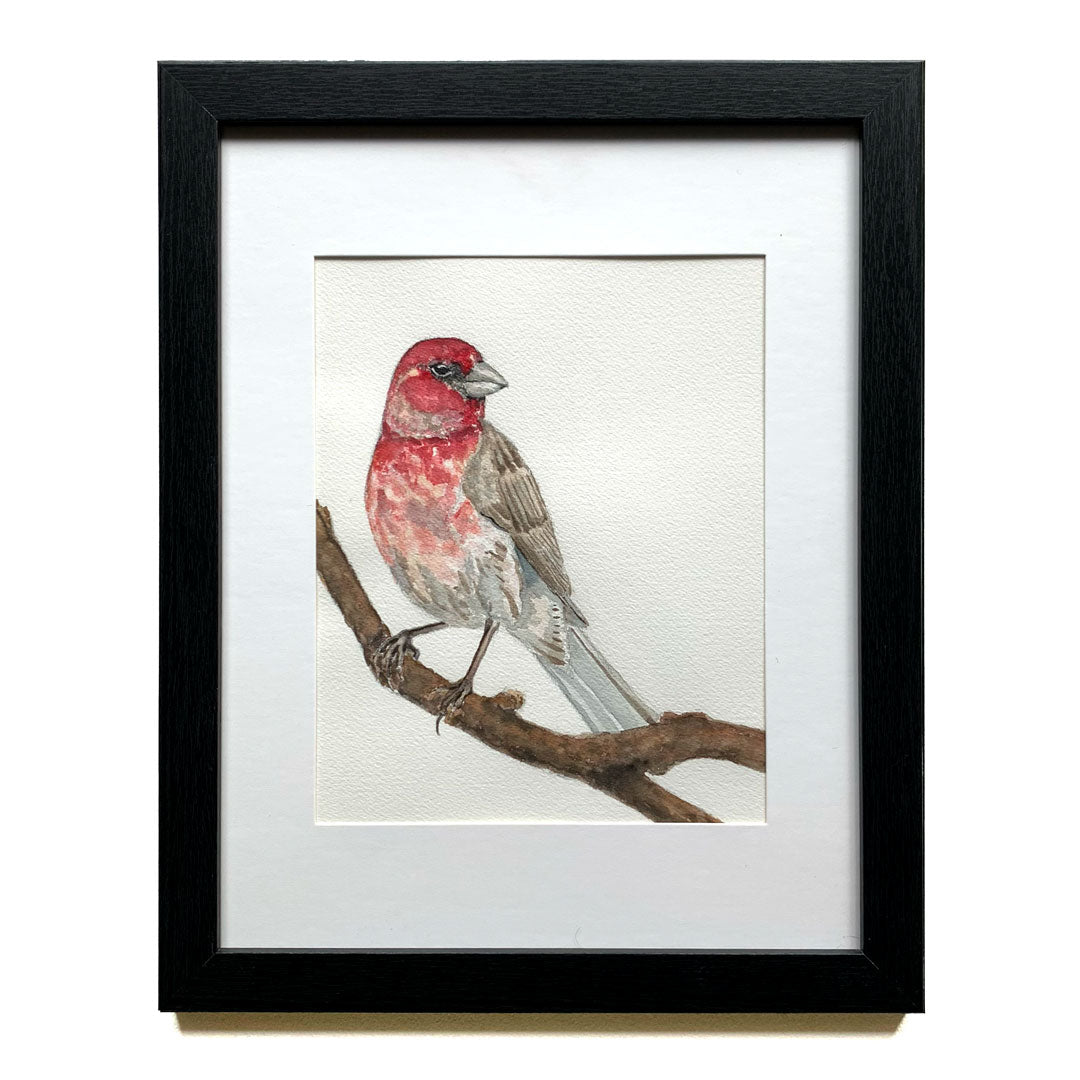This image features a framed illustration of a bird perched on a tree branch. The rectangular frame is black with a white mat, and the drawing is on a taupe or beige canvas. The tree branch, shown in light brown, runs from the middle of the canvas downward to the right and splits into two branches. The bird is a captivating blend of red, gray, and brown colors. It stands with its body facing left while looking to the right. The bird has a red head with a gray beak and black eyes. Its chest transitions from red to pink, blending into beige and gray as it reaches the lower belly. The bird's wings are predominantly gray, and its tail feathers are a lighter gray. It has dark gray legs and two gray feet that grip the branch, aiding its balance. The frame appears to be mounted on a white wall. This detailed portrayal suggests the work of a skilled local artist.